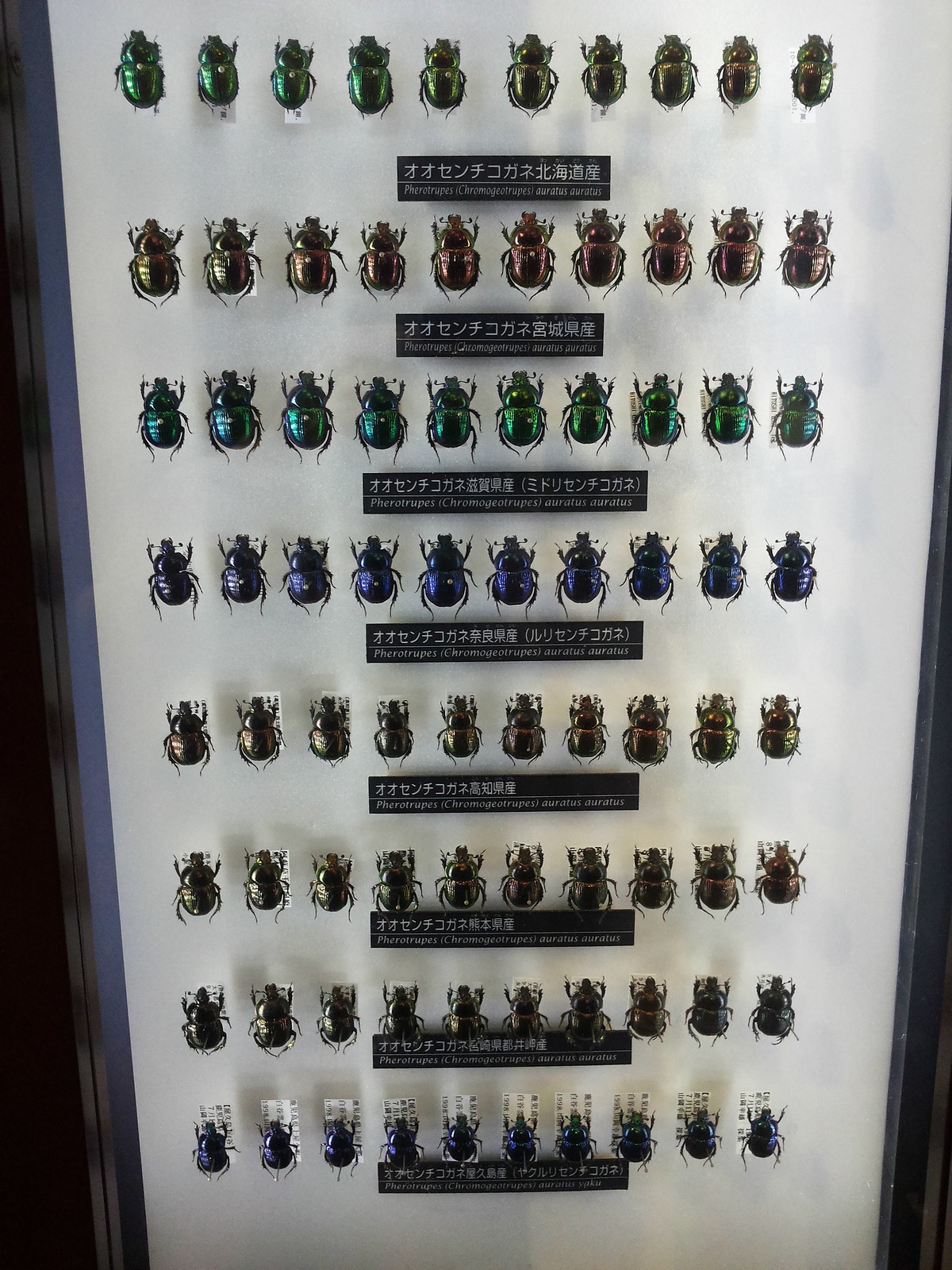This is a detailed color photograph of a framed display case showcasing 80 beetles, meticulously organized in ten rows against a white photo mat. Each row contains ten beetles, and they appear to be categorized by color. The top row features green beetles, followed by a brownish row, then green, blue, brownish again, and two rows of black beetles, culminating in a blue row at the bottom. Each row is accompanied by a small label written in either Chinese or Japanese, which likely identifies the species but is not readable. Some beetles exhibit subtle iridescent hues, ranging from green to blue and even a brassy tone. The frame of the display is black, and there are some reflections of the insects' shadows on the mat, adding a sense of depth to the composition. A hint of blue is visible along the edge to the right, framing the meticulously presented collection.